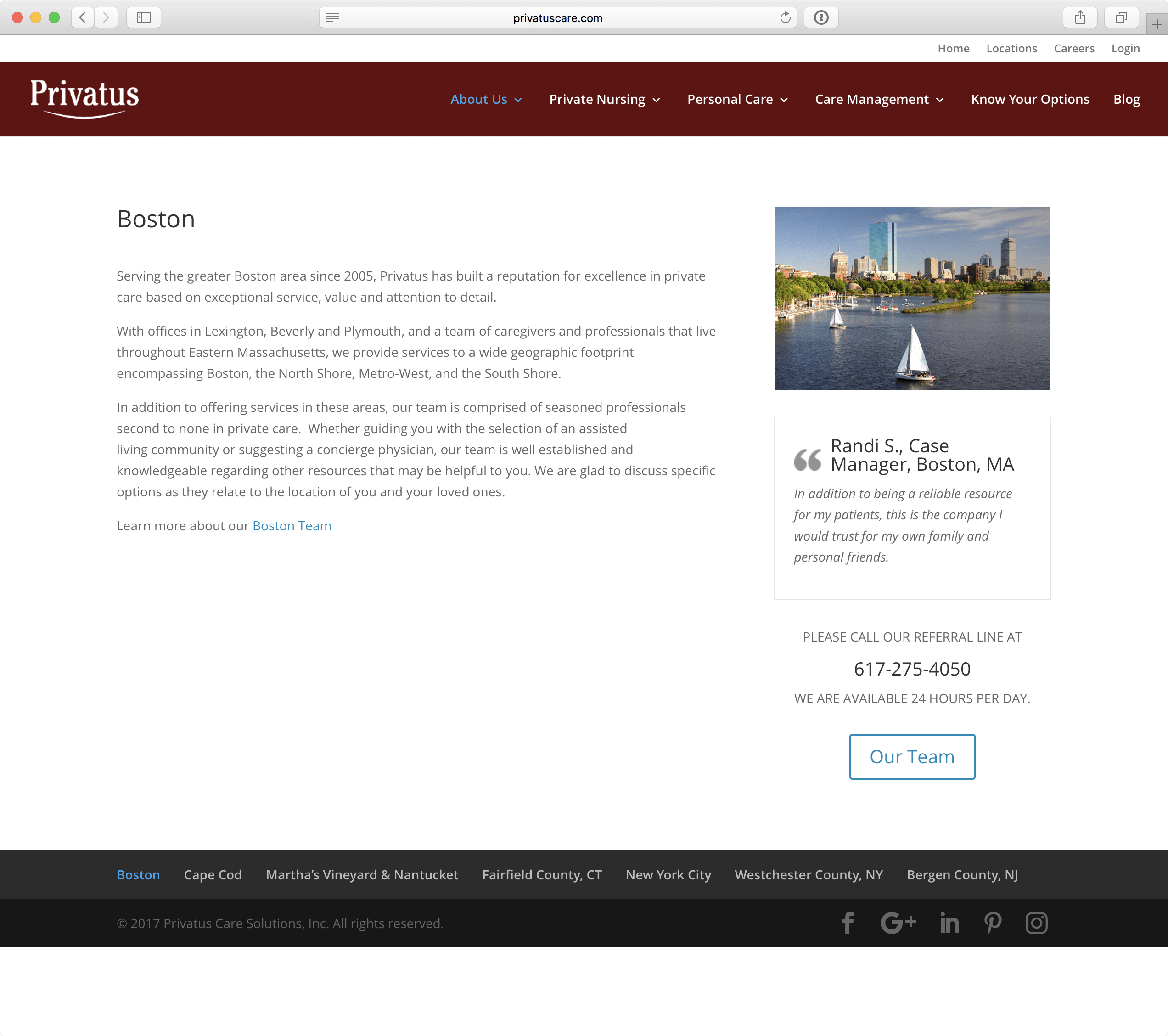The image features an interface with a distinct URL bar at the top, though its content is indiscernible due to its small and blurry nature. On the left side of the URL bar, there are three colored circles: red, yellow, and green. Directly below, there is a brownish-red navigation bar displaying "Privatus" on the left, followed by menu options: About Us, Private Nursing, Personal Care, Case Management, [Something] Option, and Blog. 

A photograph showcasing a city skyline with water and sailboats beneath it is the main centerpiece of the page. The city is identified as Boston, as indicated by the text "Boston," beneath which there are three paragraphs of text that are illegible owing to their small size. Below this text, a label reads “Randy S., Case Manager in Boston, Massachusetts.”

At the bottom area of the image, there is an "Our Team" section, followed by several social media icons for Facebook, Google+, LinkedIn, Instagram, and Pinterest.